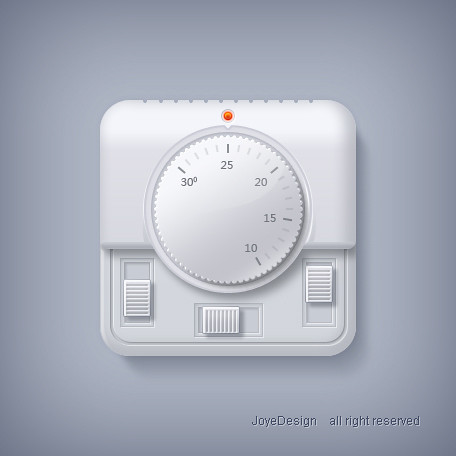The image is of a white square device resembling a thermostat, set against a gray background. The bottom right corner of the device is inscribed with the text, "Joy Design, All Rights Reserved." The centerpiece of the device is a circular dial, which is marked with a scale ranging from 10 to 30 degrees, or possibly minutes, suggesting it might function as a timer. The dial is designed to be adjustable by turning it, and features a small red dot at the top, likely indicating a light or an operational marker. Below the dial, there are three adjustable slide switches—two arranged vertically and one horizontally—allowing for various settings to be modified by sliding them up, down, or sideways. At the very top of the device, small, evenly spaced vents are visible, hinting at a possible ventilation function or additional sensory components.